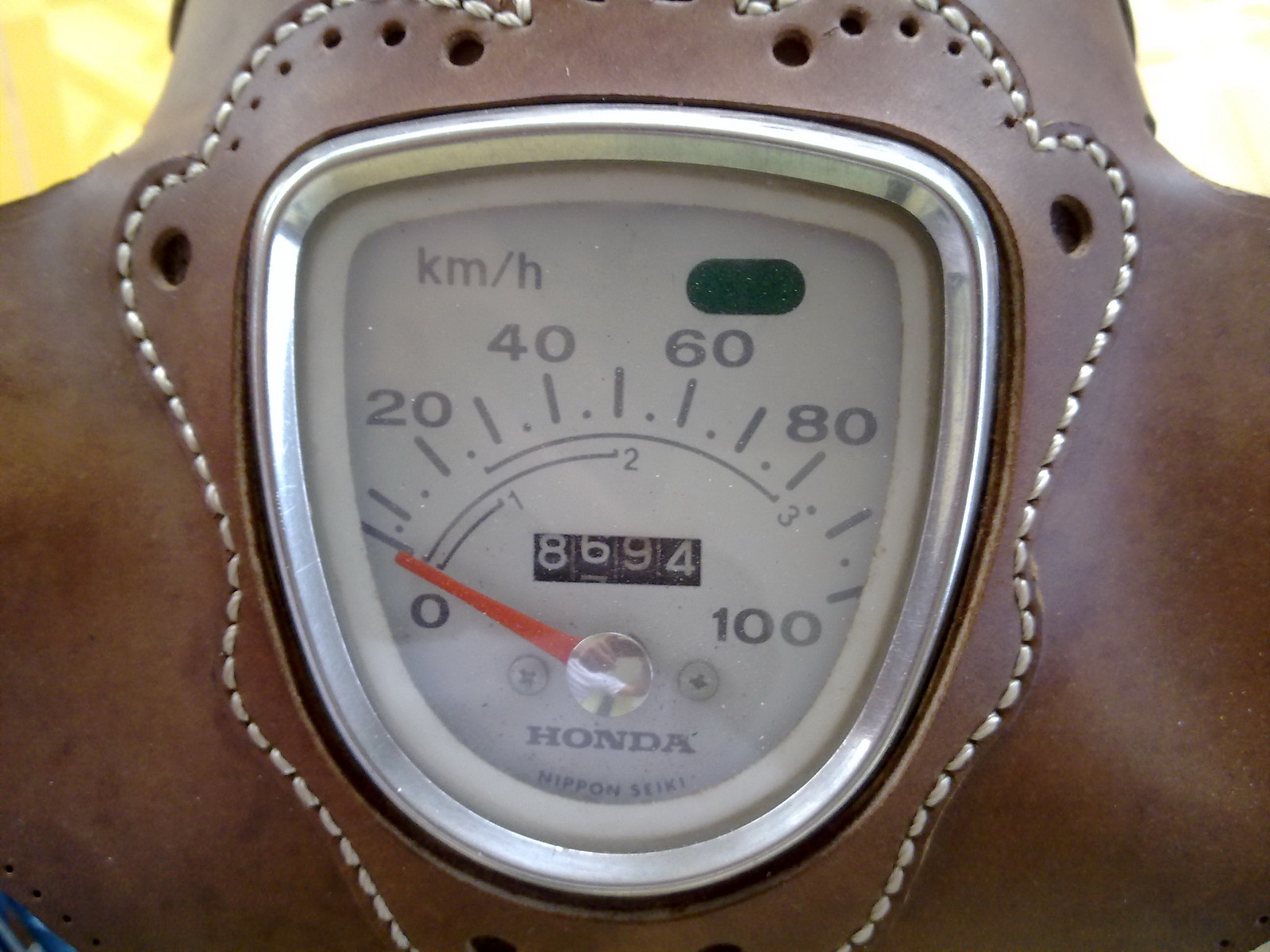In this image, we observe a detailed close-up of a classic motorcycle speedometer mounted on a piece of dark leather. At the center of the speedometer, there's a rounded triangle outline in chrome. The upper left corner of this chrome placard features the inscription "KM/H," indicating that the speed is measured in kilometers per hour. Toward the lower part of the triangle, the word "Honda" is prominently displayed, followed by "Nippon Seiki" beneath it, both hinting that this speedometer belongs to a Honda motorcycle and was manufactured by Nippon Seiki.

The speedometer dial itself presents a vintage aesthetic with a red needle resting at zero. The numeric range on the dial extends from 0 to 100 kilometers per hour, marked at intervals of 20, 40, 60, 80, and ultimately 100. Within this arc, there is also an odometer that utilizes white flip-style numbers on a black background, reminiscent of older mechanical clocks. The odometer currently reads 8694 kilometers, suggesting that this motorcycle has traveled that distance.

Additionally, beside the main speed indication arc, smaller arcs are marked with the numbers 0, 1, 2, and 3. These arcs represent the suggested speed limits for different gears: first gear can reach up to 25 km/h, second gear can reach up to 50 km/h, and third gear can extend up to 80 km/h, implying a progressive speed increase across gears.

Overall, the image provides a nostalgic glimpse into the speedometer of a vintage Honda motorcycle, offering insights into both its current mileage and its functional speed capabilities across different gears.